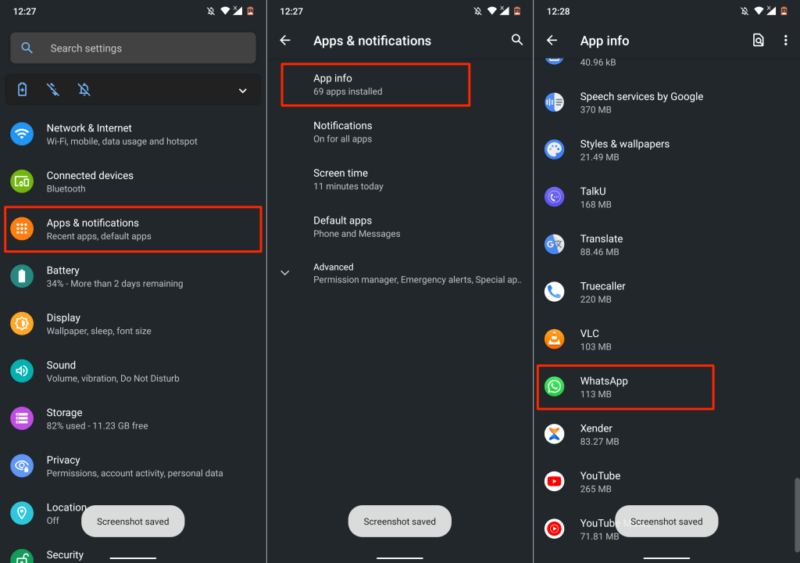A collection of three screenshots captured on a gray background at 12:27 PM, showcasing the search settings and various system panels on a mobile device. 

1. **First Screenshot:** At the top, the time is displayed as 12:27 PM alongside a search bar and a magnifying glass icon in blue. Below this, several categories are listed: "Network & internet" including Wi-Fi, mobile data usage, and hotspot options; "Connected devices" with Bluetooth settings; "Apps & notifications", which is highlighted with a red rectangle; followed by "Battery", "Display", "Sound", "Storage", "Privacy" and "Location", which is turned off. At the bottom of the screenshot is a white oval with gray text indicating the option to save screenshots.

2. **Second Screenshot:** The time shown is 12:27 PM again. The header includes a left arrow and the title "Apps & notifications," with a magnifying glass icon. The red rectangle now highlights "App info," indicating there are 69 installed apps. Other options listed are "Notifications," "Screen time," "Default apps," and "Advanced."

3. **Third Screenshot:** The time transitions to 12:28 PM, reflecting a slight passage of time. A search bar and three vertical dots for additional options are visible at the top. Below, a list of apps is displayed along with their storage usage: "Speech Services by Google" (370 MB), "Styles & wallpapers" (21.49 MB), and "TalkU" (168 MB), each app title prominently displayed in its respective entry.

The screenshots are similar in style with common elements such as the device's time, search functionalities, and navigation arrows, capturing various system configuration menus and app details comprehensively.